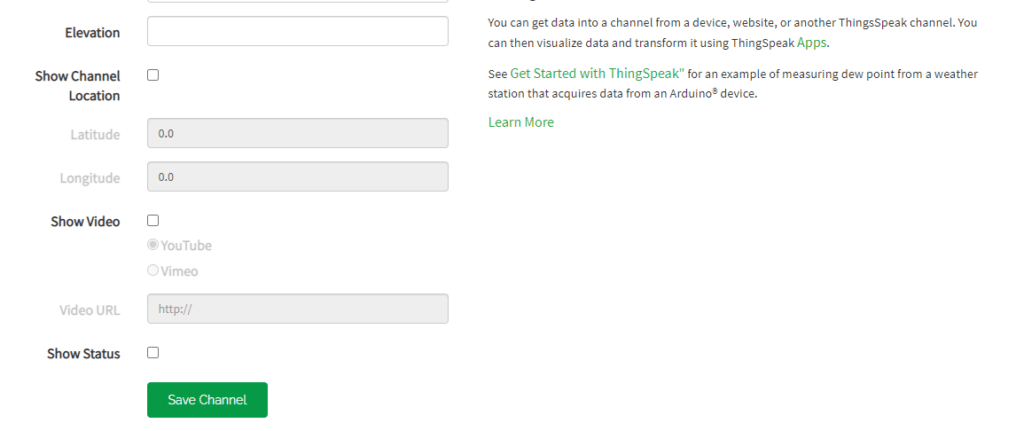"This image illustrates the process of setting up a new data channel in ThingSpeak. The user interface displays a panel with a white background and seven different input options. These inputs allow users to configure settings for acquiring and visualizing data from various sources, including devices, websites, and other ThingSpeak channels. 

For example, the interface includes options to input elevation and channel location, with the latitude and longitude fields left in gray when not specified. There are also settings to embed videos from YouTube or Vimeo, indicated by unchecked and checked boxes, respectively. The video URL input field is represented by a gray bar labeled 'HTTP.'

Additionally, there is an option to display the channel's status, which remains unchecked. To finalize the setup, a gray rectangle button labeled 'Save Channel' is shown.

On the screen, the text 'Get started with ThingSpeak' guides users through the process, emphasizing that ThingSpeak allows for the visualization and transfer of data acquired from various sources, such as weather stations using Arduino devices to measure dew point."